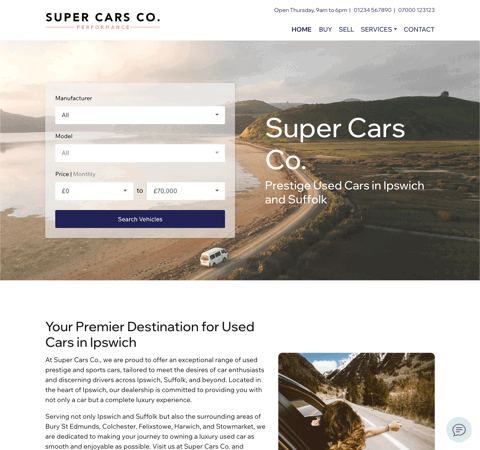This image is a screenshot of the Super Cars Company website. At the top, the site prominently displays the company’s name, "Super Cars Co.", followed by the tagline "PERFORMANCE" in smaller, red, capital letters. Below this headline, the website features "Super Cars CO" in large font, accompanied by the location "Used Cars in IPSWICH."

The main section showcases a user-friendly interface with drop-down menus where users can select a car manufacturer, model, and price range. Currently, both the manufacturer and model fields show "All," while the price range spans from £0 to £60,000. Beneath these options is a clickable rectangular button labeled "Search Vehicles."

In the background of the website, there's a photograph featuring a picturesque landscape. To the left, a watery area is visible, while large hills and mountainous terrain dominate the right side. A white minivan is driving down a road that cuts through this scenic vista. Additional text at the bottom of the screen reiterates the "Used Cars in IPSWICH" location and includes a couple of descriptive paragraphs about the dealership.